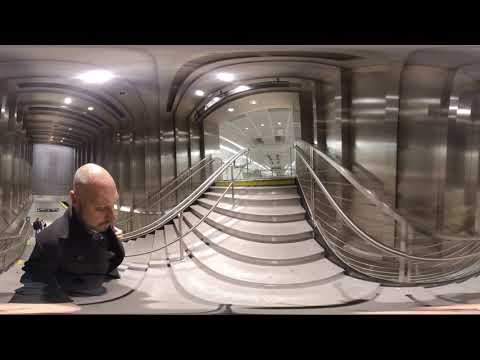The image depicts a heavily distorted panoramic shot of a modern, metallic office building featuring a staircase with metal railings and a series of lights on the ceiling. The staircase, consisting of seven or eight semi-circular steps, leads up to a distant white door. The ceiling, which appears to be made of glass and arches to create an almost spaceship-like effect, further enhances the sci-fi ambiance. To the left of the picture, a bald man, aged possibly in his 30s or 40s, with a thin beard and mustache, dressed in a black coat and pants, stands partially 'smushed' due to the panoramic distortion. His body and legs appear unnaturally short, as if caught in a time warp. The overall effect of the distorted perspective is surreal, almost as if the scene is split, contributing to a futuristic, otherworldly atmosphere.